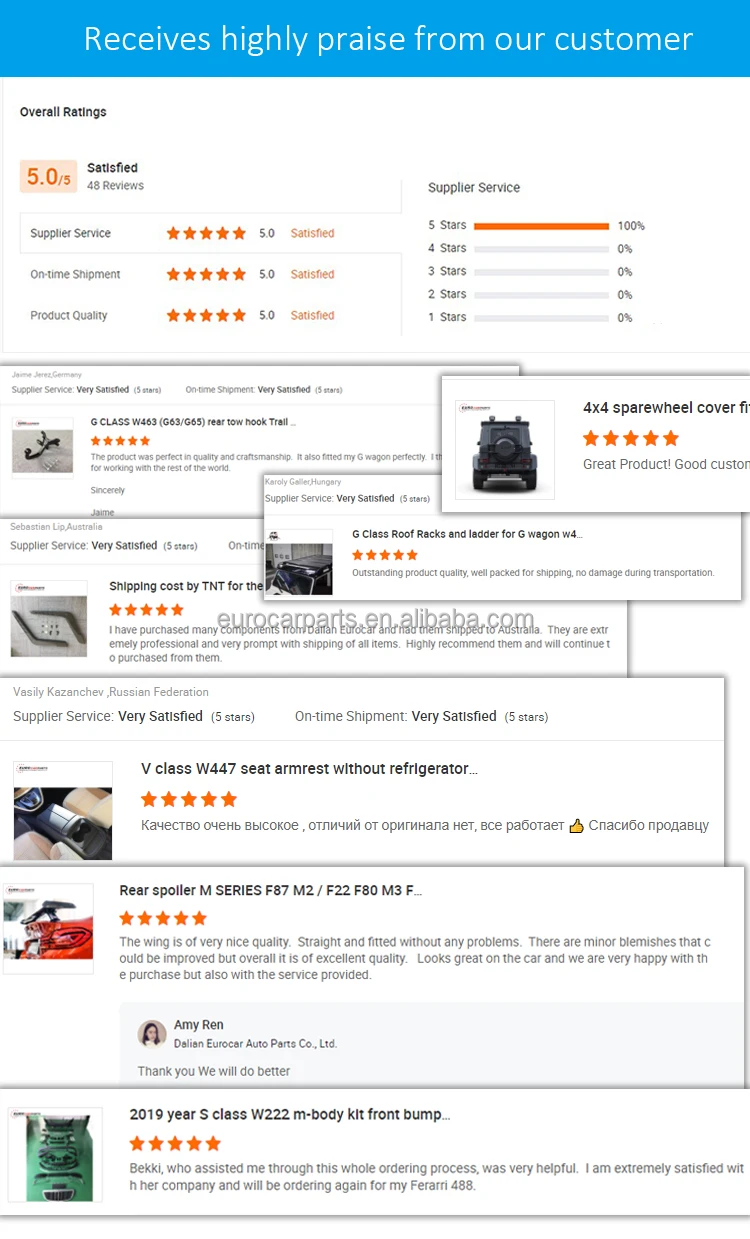The image appears to be a webpage showcasing product ratings and reviews. At the top, there is a blue banner with white text that reads "Receives highly praised from our customer." Below the banner, there is a section displaying a rating scale, indicating an overall rating of 5.0 with 46 reviews. The scale suggests that being highly satisfied equates to a 5.0 rating.

Immediately beneath this section, there are three highlighted reviews, all rated with five stars, although their specific contents are not legible. The central part of the image features a collage of seven customer reviews with respective product images. Each review block contains a product image, the review title, the star rating, and a brief explanatory text regarding the customer's experience.

The arrangement starts with the first five reviews placed in a vertical sequence, one directly below the other. The last two reviews overlap slightly with the preceding ones to ensure readability. Each review includes a few sentences, some of which are signed off with the reviewer's first and last name, adding a personal touch and authenticity to the feedback.

Overall, the image captures a well-organized display of customer satisfaction, backed by visually detailed product reviews and high ratings.